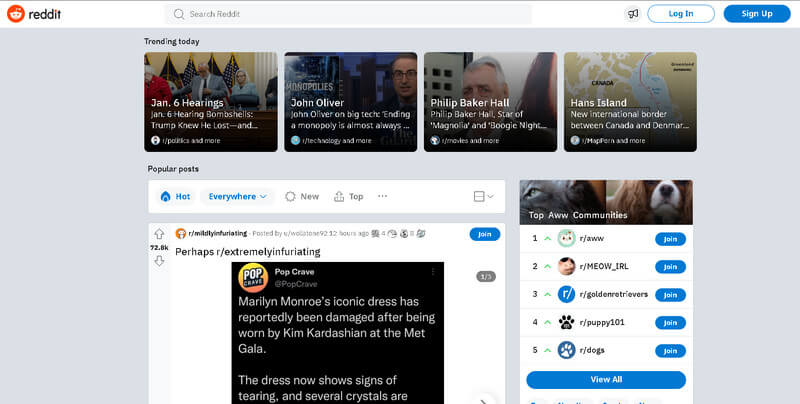The image depicts a webpage from the popular social media platform, Reddit. In the top left corner, the recognizable Reddit logo is prominently displayed, featuring a stylized red circle with a simple, smiling face inside it, accompanied by the name "Reddit" in a dark grey font with an orange dot above the "i".

At the top center of the screen, opposite the logo, is a search bar for navigating the site. To the right of the search bar, there are options to log in or sign up for an account if one hasn't been created yet.

Directly below the header, four featured images with brief text blurbs are visible, showcasing trending topics and recent discussions or news events. Among these popular posts, a notable entry highlights a discussion about Marilyn Monroe's iconic dress, which has reportedly been damaged after being worn by Kim Kardashian at the Met Gala.

On the right side of the screen, a list of top communities on Reddit is shown, inviting users to join these vibrant, topic-specific groups. There's also an option to "View All" to explore additional communities.